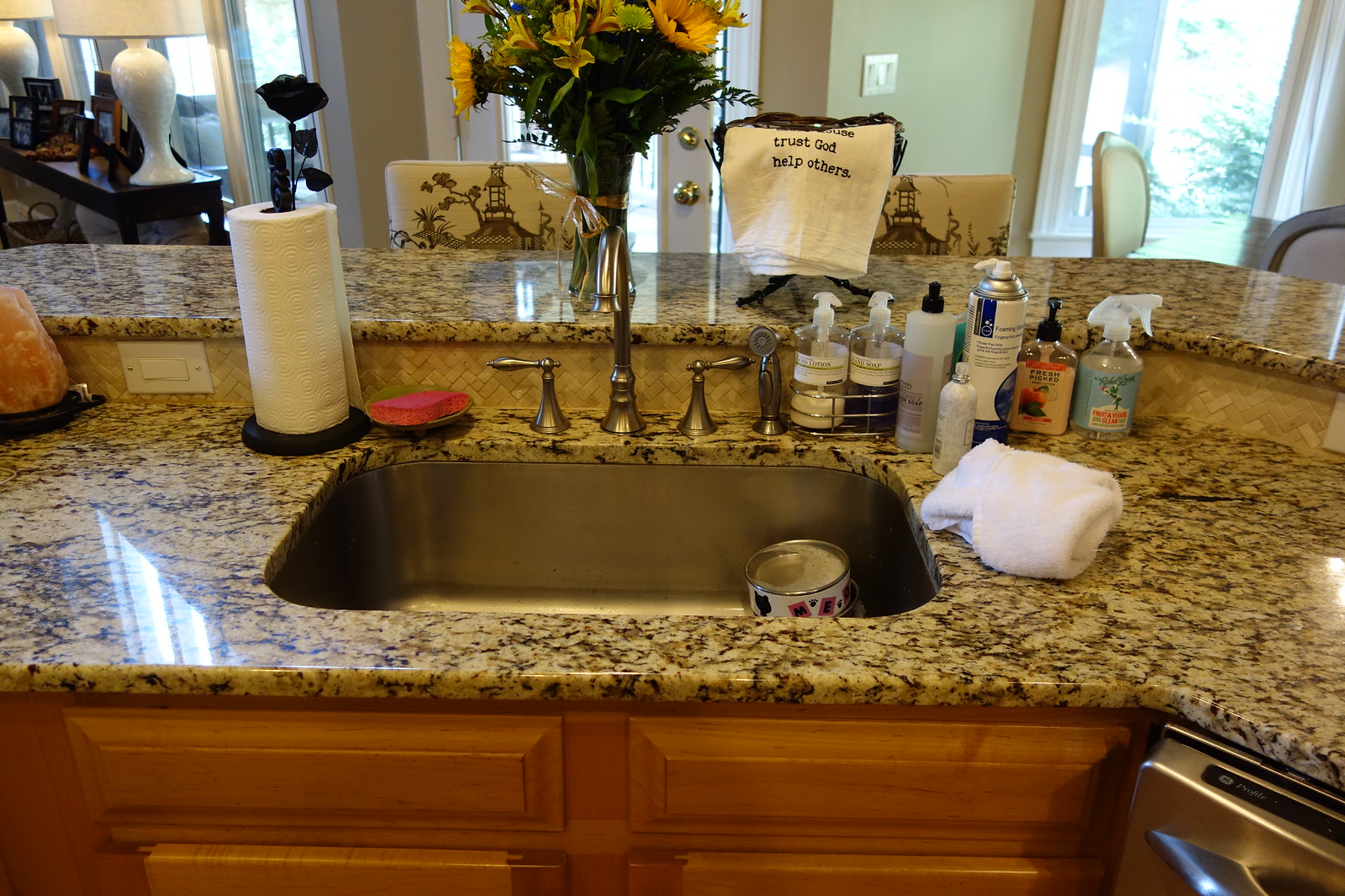The image depicts a well-used and homey kitchen space. Dominating the foreground, an island with a sleek granite countertop and built-in metal sink serves as the focal point. A silver faucet rises prominently above the basin. To the left of the sink, a standing paper towel holder dispenses a roll of white paper towels, while an assortment of soaps and cleaning supplies clutter the countertop nearby, reflecting a busy but tidy household. A cloth linen hand towel hangs casually close to the sink, adding a soft, domestic touch. Inside the sink, an empty can—its specific contents indiscernible—rests, perhaps waiting to be rinsed and recycled. Brightening up the kitchen, a small bouquet of flowers adds a splash of color to the scene. In the backdrop, the outline of a door and multiple windows suggests a continuation of the cozy, lived-in home. This image captures the everyday essence of a family's kitchen, complete with practicalities and warm details.